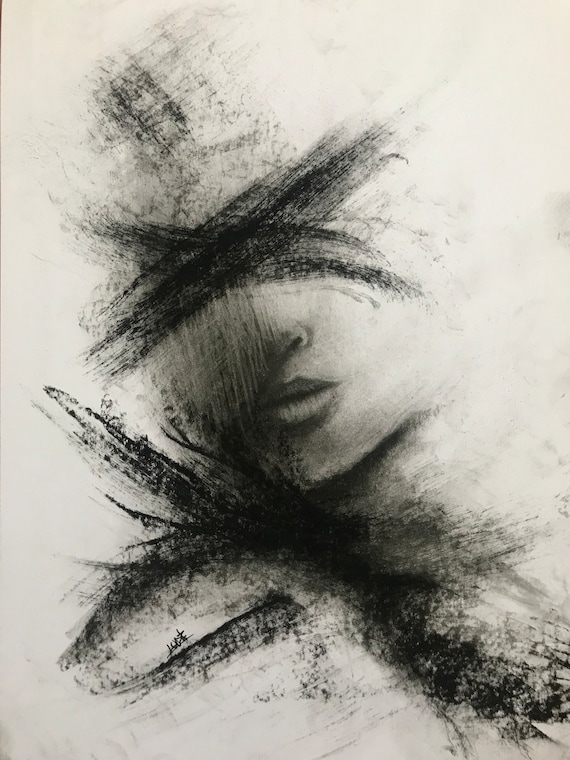In this hand-drawn charcoal artwork, presented in black and white, a partial portrayal of a woman's face emerges from a stark, light-colored background. The drawing meticulously captures her chin, lips, and one nostril of her nose, but above the bridge of her nose, an X-shaped smear of dark charcoal obscures where her eyes would be, giving the piece an abstract and fragmented feel. Further black strokes disrupt the area under her chin, extending across the lower part of the image and preventing any view of her neck down. Though primarily monochromatic, the background bears subtle shades of light gray or pinkish beige. The entire scene is photographed, revealing a sliver of the surface it rests on at the upper left corner, while a barely legible signature lies in the bottom left, possibly reading "JCT," adding a touch of mystery to the artist's identity.